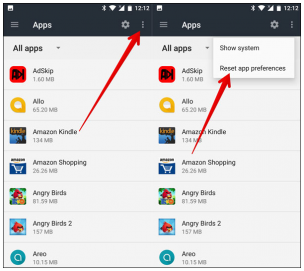This paired screenshot displays two mirrored lists of apps on a smartphone, intended to guide the user through resetting app preferences. At the top of each list, a navigation bar is visible, comprising three horizontal lines labeled 'Apps', a cogwheel icon on the right, and three vertical dots. Below this bar, the text 'All apps' appears with a downward-pointing triangle, followed by a set of apps:

1. 'ALO' featuring a red logo
2. 'Allo' with a yellow 'Q' icon
3. 'Amazon Kindle' alongside the Kindle logo
4. 'Amazon Shopping' with a shopping cart icon
5. 'Angry Birds' and 'Angry Birds 2' with their respective logos
6. 'AREO' depicted with a blue circle containing a white 'Q'

In the left screen, a red arrow points from the 'Amazon Kindle' app towards the three vertical dots. In the mirrored right screen, another red arrow directs from 'Amazon Shopping' towards an opened box showing options: 'Show system' and 'Reset app preferences' beneath it. The purpose of the images is to prompt users to tap 'Reset app preferences', clearly highlighted in the top-right corner.